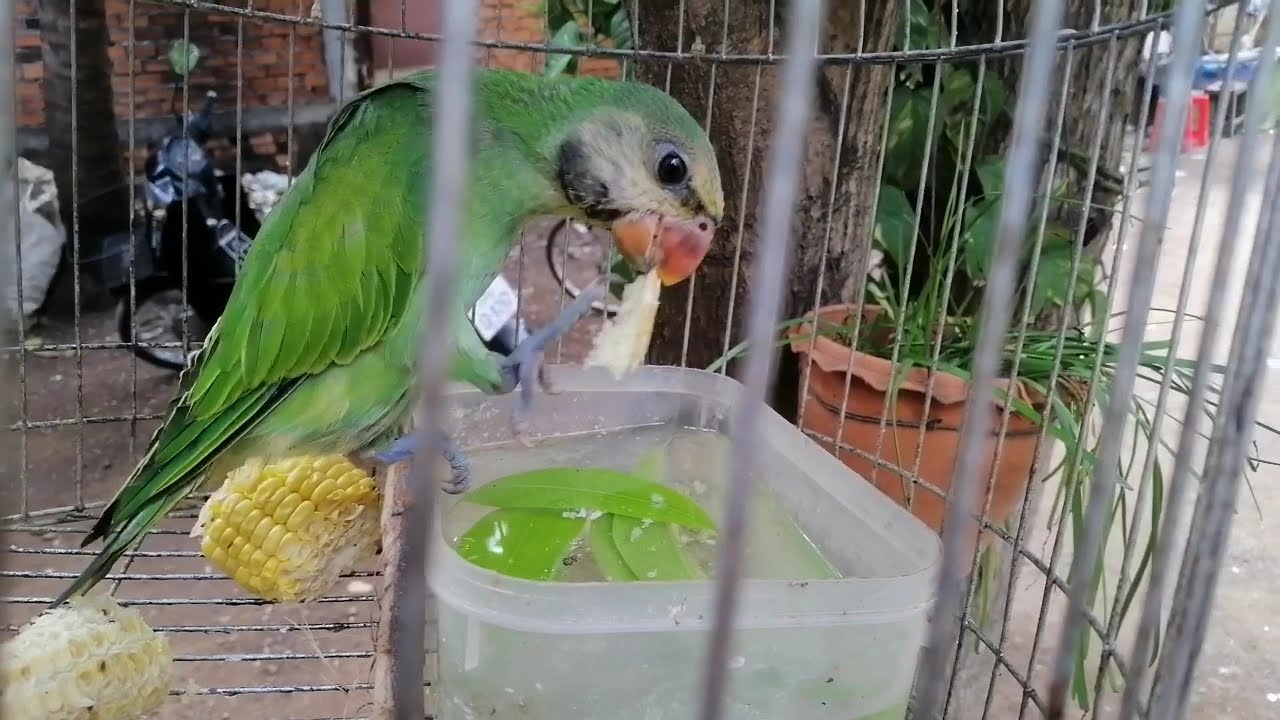In this image, we observe a green tropical parrot perched inside a silvery-gray, metal cage. The parrot, with green wings, black tail feathers, black cheek feathers, and a whitish cheek, also has a distinct orange beak. It is perched on the edge of a clear plastic container filled with water and leaves. The parrot seems to be picking at something, possibly a piece of fruit, with its orange beak and one claw reaching up to grasp it. Below the perch, there is a partially eaten yellow cob of corn. The cage is situated in an outdoor setting, evidenced by the background which features a brick wall, a motor scooter, a large tree, and a potted plant. This scene suggests the parrot is being displayed in an open, possibly public area, possibly on a street corner.